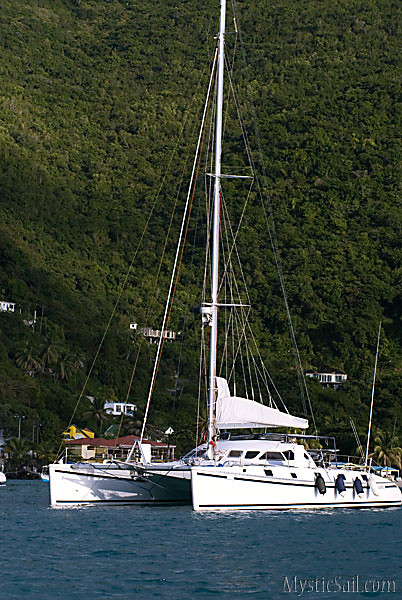The image is a serene outdoor scene set on a body of dark blue water, likely a lake or ocean, with a lush, mountainous, dark green landscape in the background. The main focus is two bright white boats, one of which is a sleek catamaran with its sails furled. Black life jackets or buoyancy devices are visible on the side of the boats. The boats stand out vividly against the blue water and green hillside, creating a visually appealing contrast. Nestled within the greenery of the hillside are four or five small houses, adding a picturesque touch to the landscape. The image is used in an advertisement for MysticSail.com, with the company's logo appearing in white print in the lower right-hand corner. The photograph is vertically oriented, being taller than it is wide, and emphasizes the grandeur of the natural surroundings and the elegance of the boats.